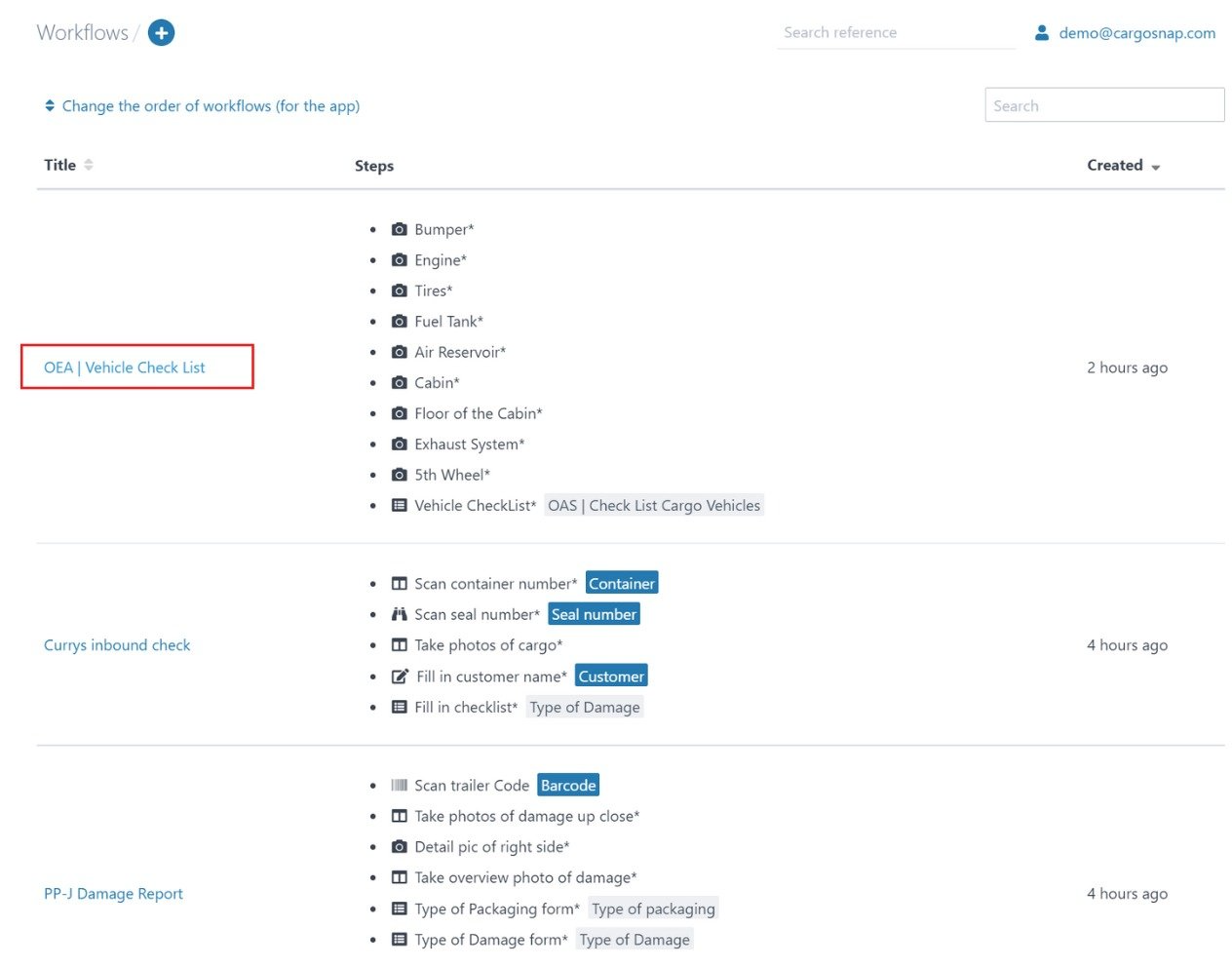The image features a clean, white background with a detailed workflow diagram. Central to the layout is a blue circle containing a plus symbol, suggesting the addition of new tasks or data. At the top, there's a search reference demo pointing to "cargosnap.com," accompanied by a functional search bar. 

The diagram demonstrates the reordering of workflows within an application, indicated by steps enclosed in parentheses. Various elements of the workflow are annotated with titles and labels. A prominent red rectangle highlights the "OEA Vehicle Checklist," listing components such as the bumper, engine, tires, fuel tank, air reservoir, cabin, floor of the cabin, exhaust system, and fifth wheel—all accompanied by camera icons.

To the left, there's a section for "Vehicle Checklist" and "OAS Checklist Cargo Vehicles," set within a gray-highlighted box. This section includes detailed steps like "Curry's Inbound Check" (highlighted in blue), "Scanned Container Number" (with 'container' in a blue rectangle), "Scanned Seal Number" (with 'seal number' in a blue rectangle), "Take Photos of Cargo," "Fill in Customer Name" (with 'customer' in a blue rectangle), and "Fill in Checklist Type of Damage" (within a gray rectangle). 

Adjacent to these steps, time allocations are provided—such as "two hours" and "four hours"—indicating the expected duration for specific tasks. Moreover, "PP-J Damage Report" is highlighted in blue, underscoring a specific part of this elaborate workflow.

Overall, the image serves as a detailed guide for a vehicle checklist and cargo inspection process, complete with visual icons, time allocations, and direct references to user interaction elements within the CargoSnap application.